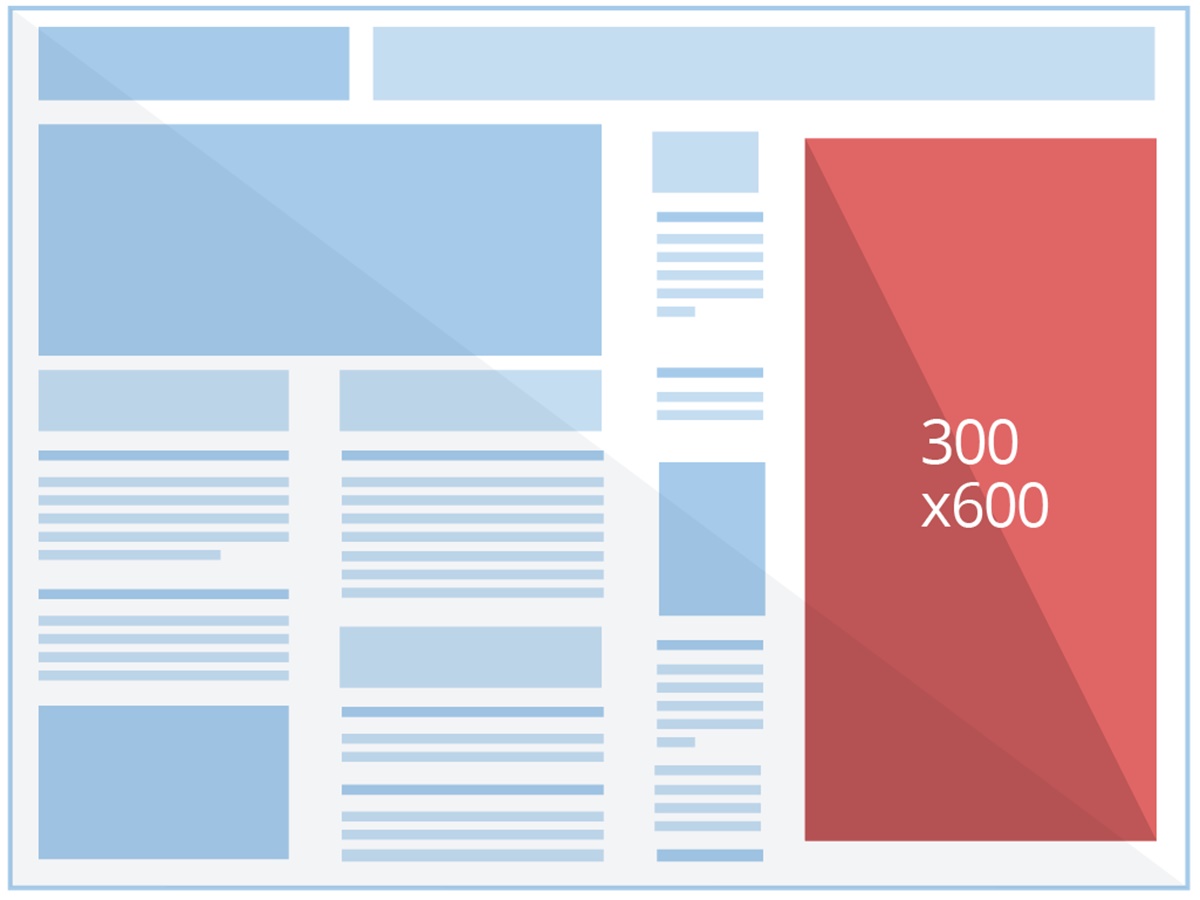The image predominantly features a collection of blue boxes and intersecting lines. On the left side of the image, there is a tall blue rectangle inscribed with the dimensions "300x600" in white text. Amid these blue elements, there is an orange, vertically oriented rectangle on the right side, which is half red and half orange, also displaying the dimensions "300x600" in white text. The intricate pattern of blue boxes and lines creates a structured, grid-like appearance across most of the image.